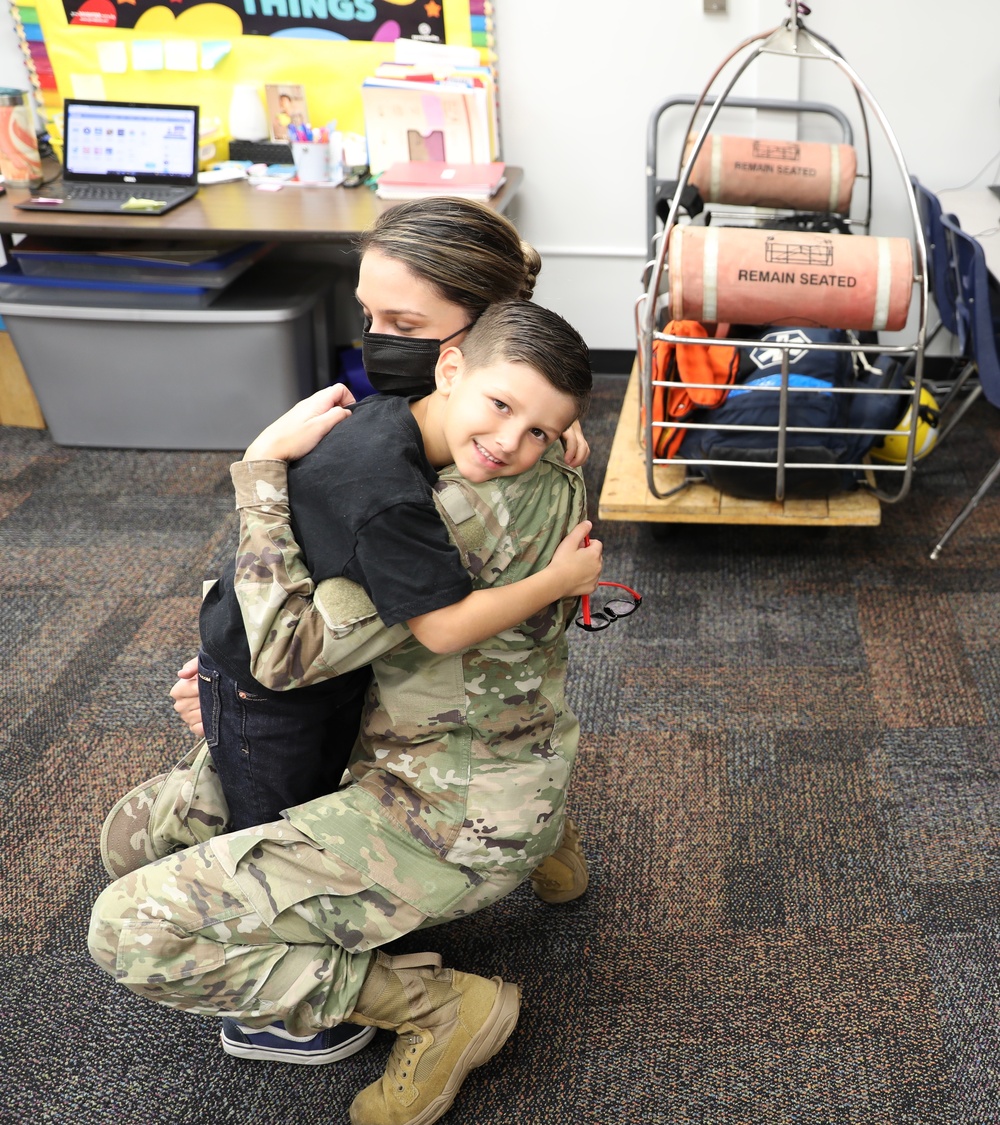This detailed photograph captures a poignant moment between a National Guard soldier and a young boy, likely her son, reuniting in what appears to be a school setting. The soldier, a woman with her hair up in a bun, is kneeling down, wearing a camouflaged uniform, brown combat boots, and a black face mask. She embraces the boy, who is smiling warmly at the camera. The boy, dressed in a black short-sleeve shirt, black jeans, and sneakers, grips sunglasses in his right hand.

The setting is a classroom, evidenced by the multicolored carpet squares and blue school chairs. To the left, there is a desk with an open laptop atop it, accompanied by various objects such as file folders, sticky notes, and a storage bin underneath. Behind them, a metal dolly filled with emergency equipment, including two inflatable life rafts labeled "Remain Seated," a yellow helmet, and life jackets, hints at the soldier's recent duties. On the wall behind the desk, children's artwork hangs from a bulletin board, completing the scene of a tender and emotional reunion amidst the backdrop of a school environment.